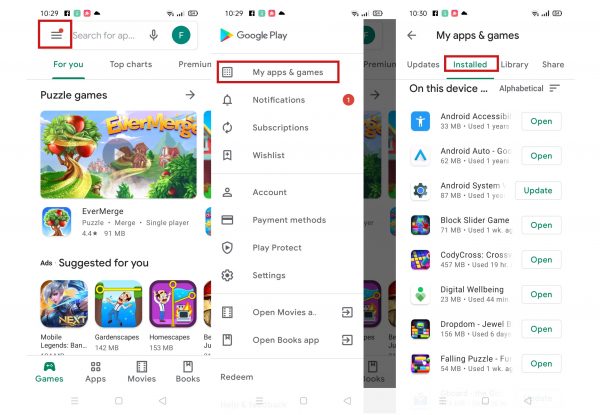This image is a composite screenshot displaying various views of the Google Play Store on a mobile phone. The screenshots are arranged vertically side-by-side.

- **Left Frame:** This view shows the homepage of the Google Play Store. At the top, there is a search bar with the prompt "Search for apps..." and a microphone icon to its right. Next to the microphone icon, there's a teal circle with a white 'F' inside it. On the left end of the search bar, there are three horizontal gray lines stacked on top of each other, which are highlighted in red with a small red dot in the top right corner. Below the search bar, several app icons are displayed.

- **Center Frame:** This view features a white sidebar overlaying the homepage. The sidebar lists several options, including "My Apps and Games," "Notifications," "Subscriptions," "Wishlist," "Account," "Payment Methods," "Play Protect," "Settings," "Open Movies" (truncated), and "Open Books App." The top option, "My Apps and Games," is highlighted with a red rectangle and accompanied by a logo resembling a gray square with gray dots.

- **Right Frame:** This view focuses on the "My Apps and Games" section accessed from the sidebar. The white sidebar that appears is labeled "My Apps and Games" and displays four options underneath: "Updates," "Installed," "Library," and "Share." The option "Installed" is highlighted with a red rectangle and shows a list of installed apps beneath it.

Each frame captures a different aspect of the Google Play Store interface, providing a comprehensive overview of its layout and navigation.